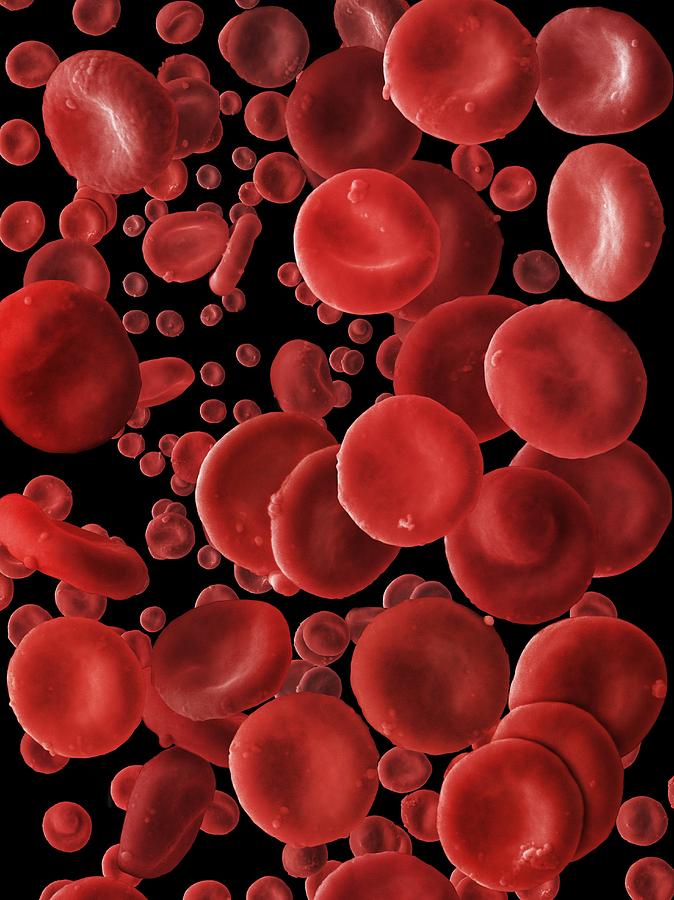This is a detailed, CGI-rendered illustration depicting an array of red blood cells floating against a stark black background. The image is densely populated with these cells, creating a vivid contrast. The red blood cells are predominantly circular with a distinctive concave shape, almost resembling jelly candies due to their glossy texture and slight indentations in the center. They vary in size and orientation, with larger and more detailed cells positioned in the foreground, gradually transitioning to smaller, less distinct ones in the background. Among the predominantly circular forms, there are a few uniquely shaped cells resembling pills, beans, hot dog buns, or cheese, adding an interesting variety to the scene. Some cells exhibit a subtle white glare, enhancing their three-dimensional appearance and highlighting the intricate CGI artistry of the illustration.